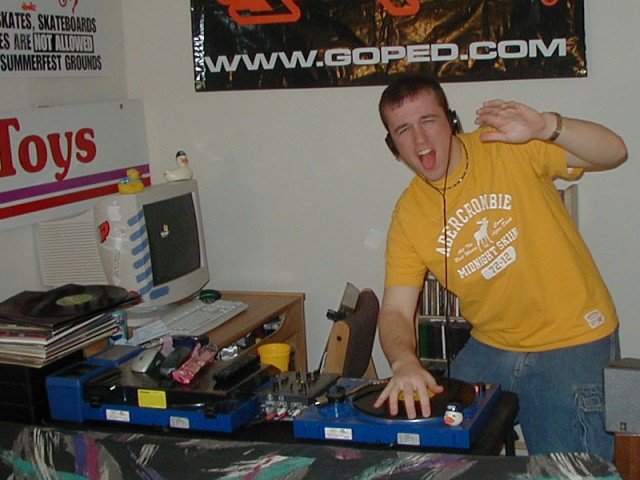The photograph captures a young man, likely a homegrown DJ, immersed in his music. He is wearing a yellow Abercrombie t-shirt and baggy blue jeans. Positioned behind a pair of black turntables with blue accents, he has one hand on a record and his other hand waving energetically above his head. He wears headphones, with his mouth open as if he's mid-sentence or singing along. 

In the background, a white wall is adorned with various posters. One prominent poster, partially visible, features the URL "www.goped.com" in white text on a black background with some red lettering obscured. Another wall displays a red-lettered poster reading "toys" and an adjacent poster with black text mentioning that skateboards are not allowed in summer fest grounds. 

The room, likely serving as his DJ corner, includes a desk behind him holding a stack of albums, a PC with a keyboard, and a screen topped by two duck figurines. The overall ambiance suggests a personal space dedicated to his passion for music.